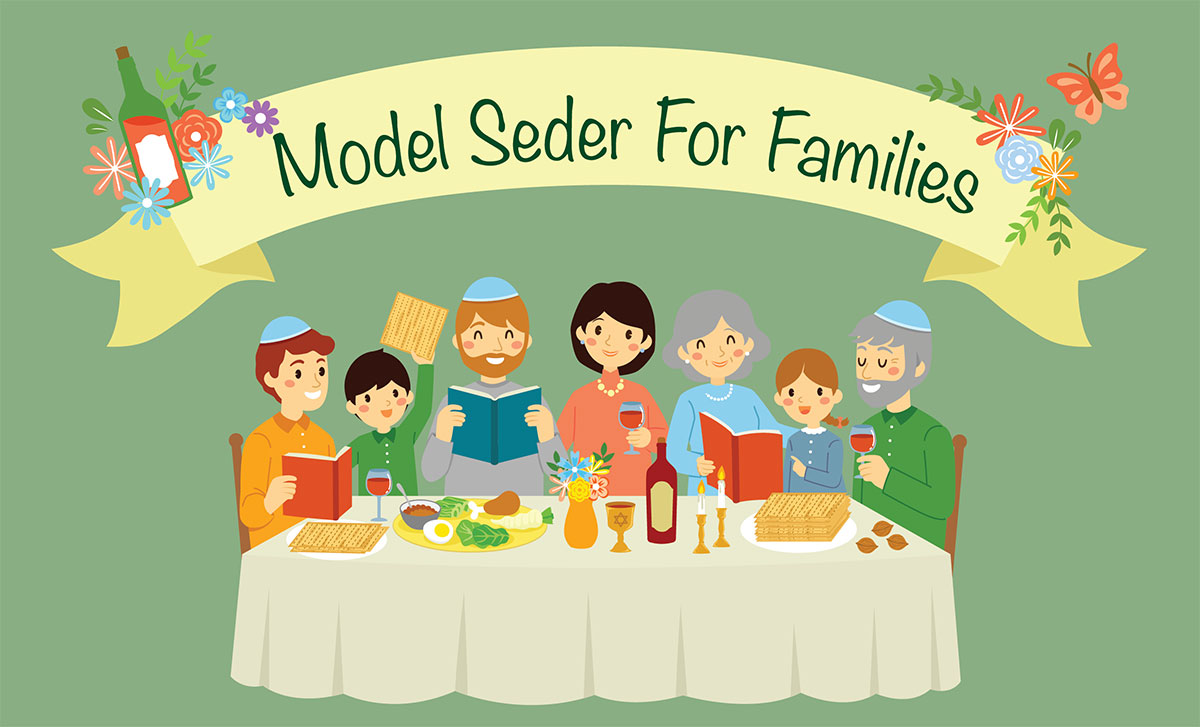The image is a detailed illustration of a Jewish family celebrating a Seder during Passover, prominently featuring a banner that reads "Model Seder for Families" in green text on a yellow background. The scene is set against a medium green backdrop with additional decorative elements including flowers, butterflies, and a wine bottle with an orange and white label at the corners of the banner.

The scene centers around a multigenerational family sitting around a long dining table covered with a beige/off-white tablecloth. Key details include:

- **Family Members:** The family includes parents, children, and grandparents. Notably, three men are wearing blue yarmulkes, indicating their Jewish faith. The individuals depicted include a little boy in an orange shirt holding a book, a boy in green with black hair without a cap, a bearded adult man holding a book, a woman in an orange dress with a glass of red wine, an elderly woman with gray hair and pearls in a blue dress holding a book, a little girl in a blue dress, and an older man with gray hair and a beard in a green shirt also with a yarmulke.
  
- **Table Setting:** The table is adorned with various elements specific to a Passover Seder, including platters of food, a vase with flowers, bottles and glasses of wine, candles on candlesticks, matzah, and possibly some cakes.

This festive and colorful illustration, with its vibrant palette of greens, yellows, grays, reds, and whites, depicts a warm and lively familial gathering celebrating a significant Jewish tradition.